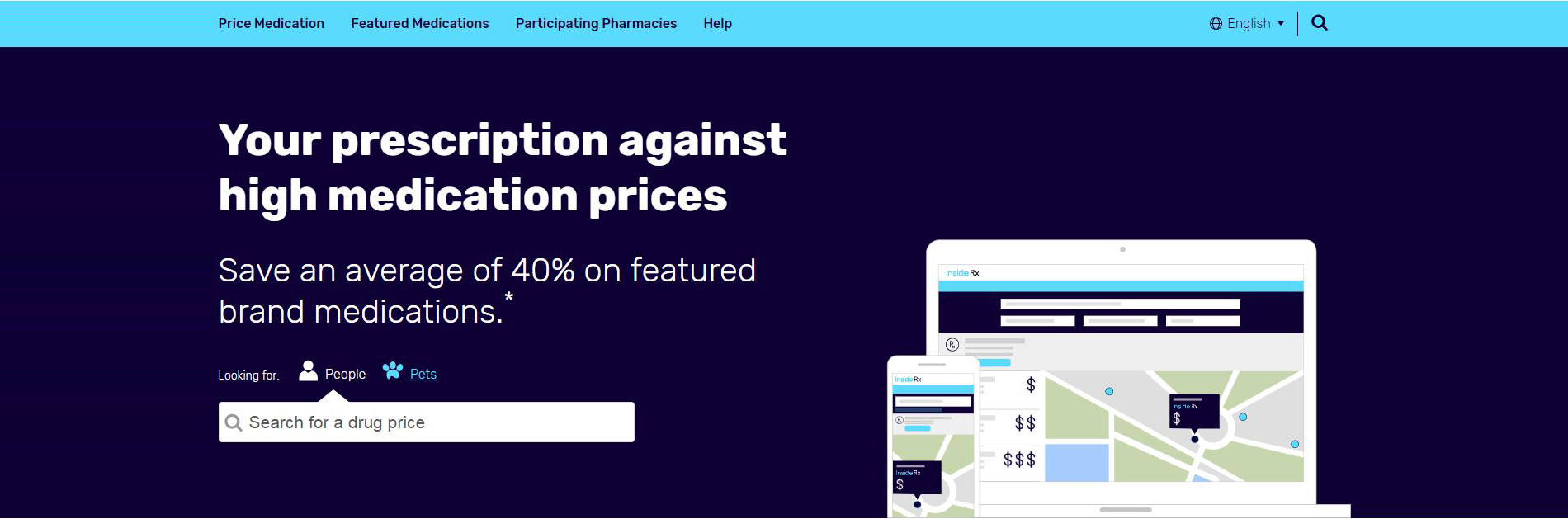This is a screenshot featuring a sleek and modern webpage designed to help users find medication prices. The top section of the screenshot is adorned with a thin, turquoise-colored border. Adjacent to this border is a menu that includes the following navigation options: "Price Medication," "Featured Medications," "Participating Pharmacies," "Help," "English," and an iconic magnifying glass representing the search function.

The main body of the screenshot has a black background, providing a stark contrast to the white text displayed prominently on the left side. The headline reads, "Your Prescription Against High Medication Prices," emphasizing the potential savings with the phrase, "Save an average of 40% on Featured Brand Medications," marked with a small white asterisk next to it.

Below this headline, the text "Looking for People" is displayed alongside a simplistic icon of a person's outline. Directly next to this, the word "Pets" is highlighted in turquoise, underlined, and accompanied by a turquoise-colored paw print icon. "Pets" is written in striking turquoise letters, making it stand out prominently.

Underneath these elements is a search bar that invites users to "Search for a Drug Price," with an upward-pointing arrow indicating the "People" category. Adjacent to the search bar, a dual illustration showcases a cell phone and a computer monitor, both displaying the same webpage. At the top of this illustration, "Inside Rx" is featured, with "Inside" in turquoise letters and "Rx" in black. Beneath the logo, there are several horizontal lines designed to simulate text content, though no specific text is provided in the illustration.

This detailed screenshot captures the essence of the webpage, highlighting its user-friendly design and functionality aimed at reducing medication costs.